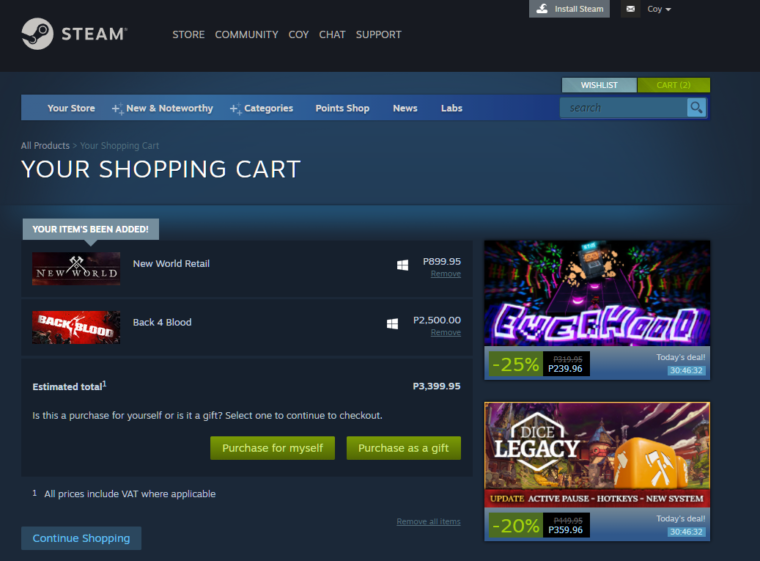The image depicts a detailed layout of the Steam digital distribution platform interface. Dominating the top section is a blue background with a prominent black box featuring a gray circle and a small black symbol that closely resembles an arm or foot. The black box prominently displays the label "STEAM" alongside navigation options: Store, Community, Koi, Chat, and Support.

On the top-right corner of the interface, there’s a noticeable grey button labeled "Install STEAM." Below that, there is an option labeled Koi, accompanied by a downward arrow. The dark blue background beneath this area encloses a lighter blue box. This inner box contains several sections titled Your Store, New and Noteworthy, Categories, Point Shop, News, and Labs. Just above these sections, a light blue box is labeled Wish List, and a green box marked Cart 2 is also visible, indicating items present in the shopping cart.

The shopping cart section lists items recently added for purchase. Featured prominently is "New World Retail" priced at $899.95. Below this, "Back for Blood" is shown with a price tag of $2500. The estimated total for these items is displayed as $3399.95. The interface then prompts the user to decide if the purchase is for themselves or intended as a gift, with green buttons labeled "Purchase for Myself" and "Purchase as a Gift" to facilitate the selection.

Towards the bottom, a small symbol resembling a "Z" accompanies the notation "All Prices Include VAT or Applicable." There is also a grey button labeled "Continue Shopping" and separated by a thin line is a section displaying thumbnail images of the ordered items for visual reference.